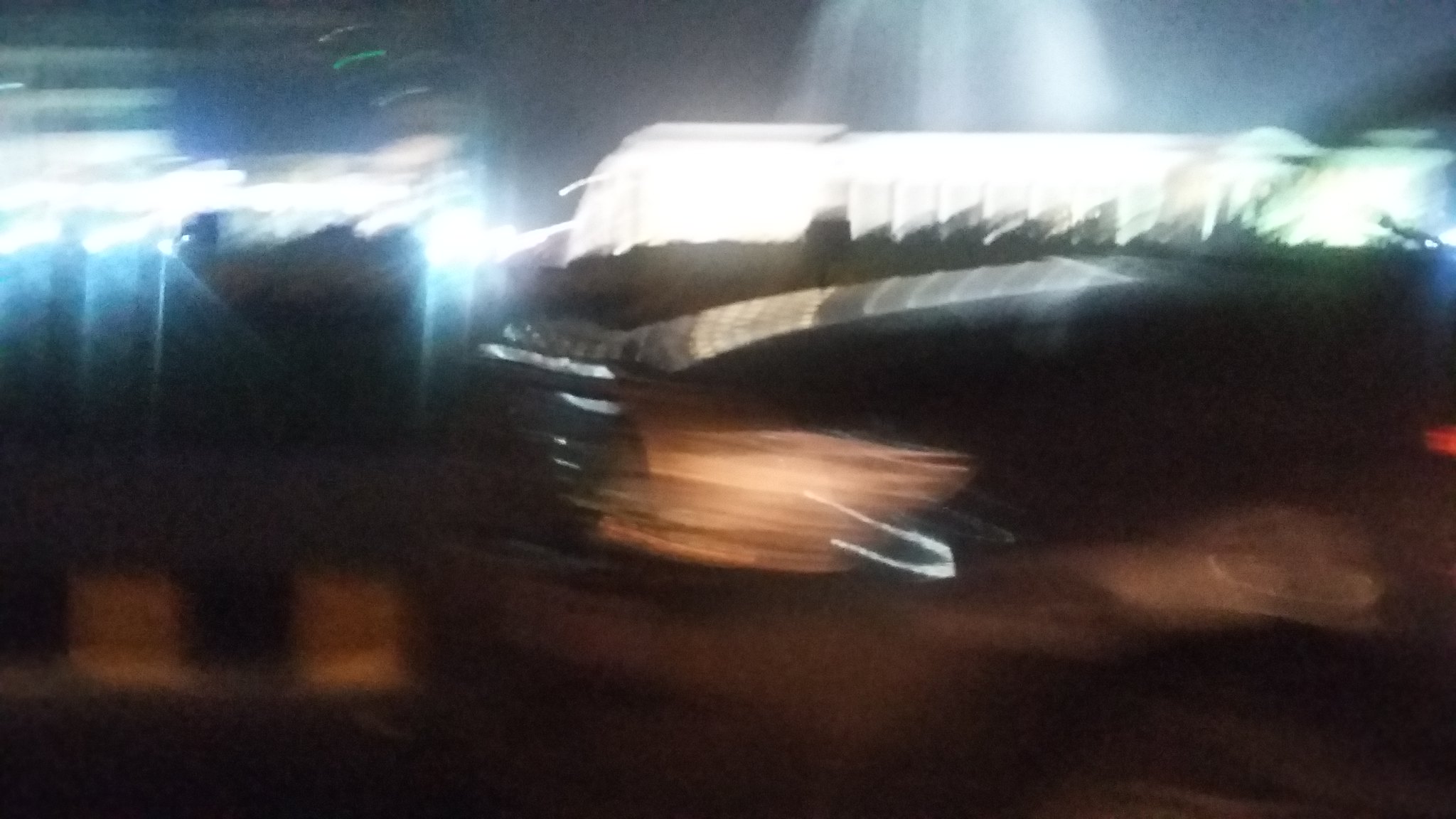The image captures a nighttime scene, heavily blurred presumably due to motion. An indistinct dark-colored vehicle, likely a truck, is traveling on a dimly lit road. The truck's yellowish headlights are clearly on, casting a low glow on its path. There appears to be a metal guardrail along the roadside with a yellow marking underneath, confirming its function as a barrier. The scene also features a lot of bright lights on the left side, potentially from light poles emitting a whitish-blue hue. These lights might be illuminating a building that doesn’t have its own lights on. Behind the truck, there's another structure or brightly lit decoration adding to the scene's nighttime vibrancy. The road, likely divided by yellow and black bars, hints at lane separation, and small details in the image suggest a backdrop of urban elements in motion.